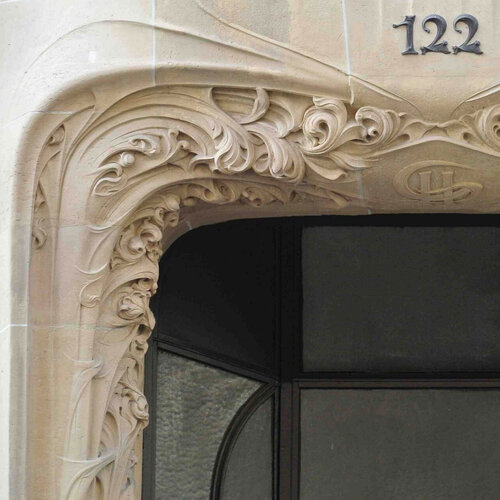This is an up-close photograph of an ornate front door. The doorway belongs to a light cream-colored building with a hint of peach. In the upper right-hand corner, the number 122 is displayed in black or dark grey. Surrounding the numbers, the doorway frame is decorated with intricate carvings that depict leaves and possibly a tree blowing in the wind, resembling cobblestone or cut stone with a highly detailed design. Additional ornate elements like round scrolls, flowers, and ivy can be seen around the frame. At the center top of the doorway, the initials CH are prominently etched into the design. The door itself features opaque white glass panes framed by dark black metal, adding to the overall elaborate and decorative nature of the entryway.